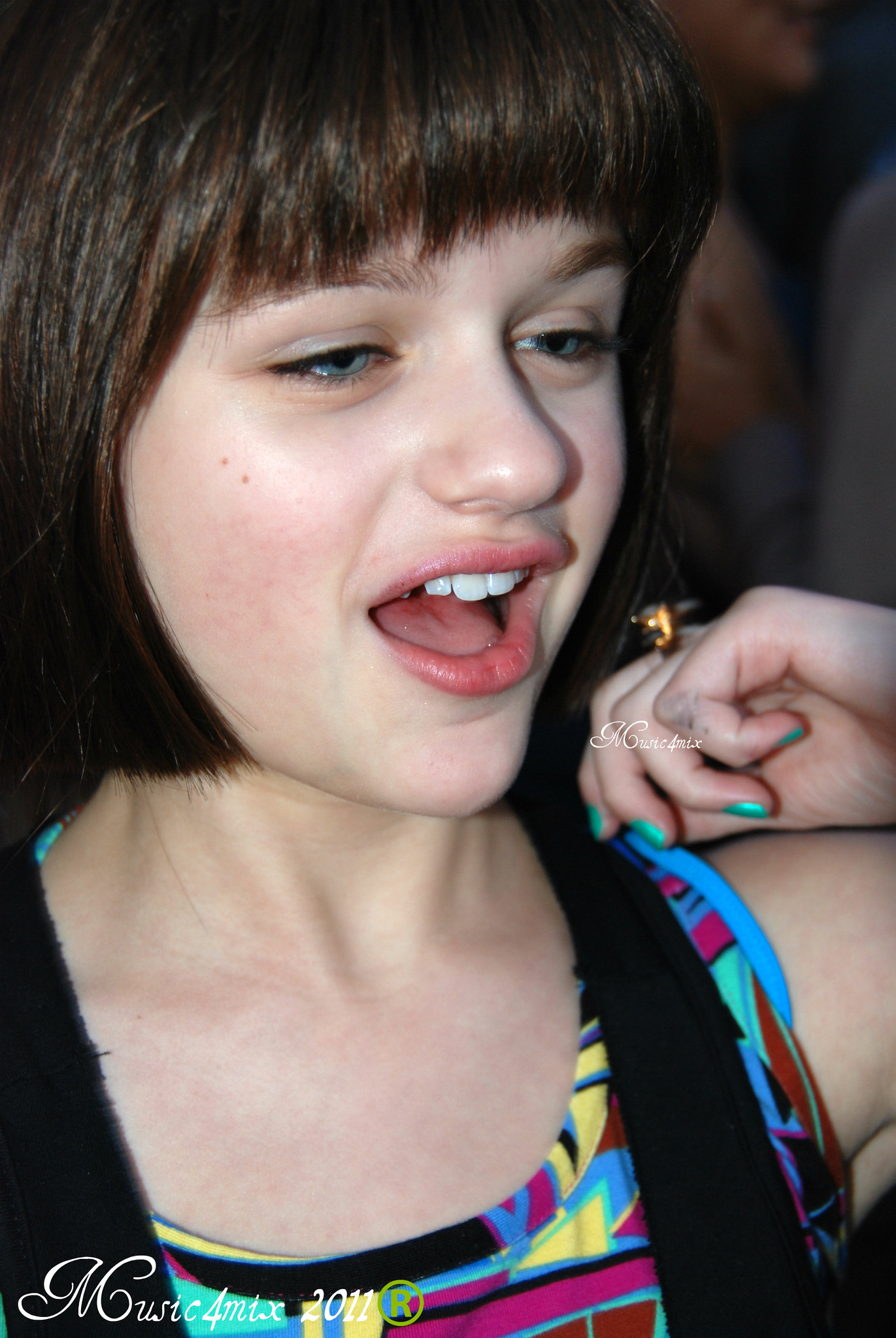The image is a close-up color photograph of a young woman in her late teens or early 20s, positioned in the bottom left of the frame. She has dark brown hair styled in a short bob cut that is cropped at the chin, though part of the back and top of her head are cut off by the edges of the image. The woman is looking or speaking towards the right, with her mouth slightly open. She has light-colored blue eyes.

She is wearing a sleeveless, multicolored tank top covered in various geometric shapes in shades of yellow, purple, pink, blue, and dark red. Black straps around her shoulders suggest she is carrying a backpack or bag. Her right hand is held close to her mouth, fingers slightly curled and her nails painted a greenish-blue hue. A large gold ring adorns one of her fingers, and there is a small black smudge on her pinky finger.

Overlaying the photograph in the bottom left corner, there is white cursive text that reads, "Music for Mix 2011." Additionally, a giant "R" in green text is prominently displayed. The overall style of the image is photographic representationalism realism.